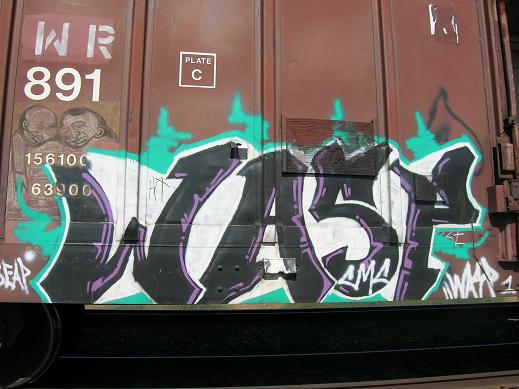This detailed landscape-oriented color photograph captures the side of a rust-colored, reddish-brown railroad car, which fills the entire image except for a black strip along the bottom. The car is marked with various stickers and white notations on the left side, including the sequence "WR 891 156 100 639 900" and an outlined white square with "plate C" inside it. The majority of the attention, however, is drawn to the vivid graffiti that stretches across the bottom half of the car, occupying the full width of the image. 

The graffiti prominently features the word "WASP" in large, black letters intensified with light purple accents and teal, or aqua blue, squiggly lines in the background. Additionally, a cartoon sketch of two people appears on the upper left side of the word "WASP," accompanied by the numeric notation "891." A white drop shadow enhances the lettering, adding depth to the graffiti. There is also a small signature tag bearing the initials "LMA" on the "S" and another instance of the word "WASP" in white graffiti-style lettering at the bottom right corner. The overall style of the image captures a blend of photographic realism and representational artistry, showcasing the dynamic and layered street art on the train car.